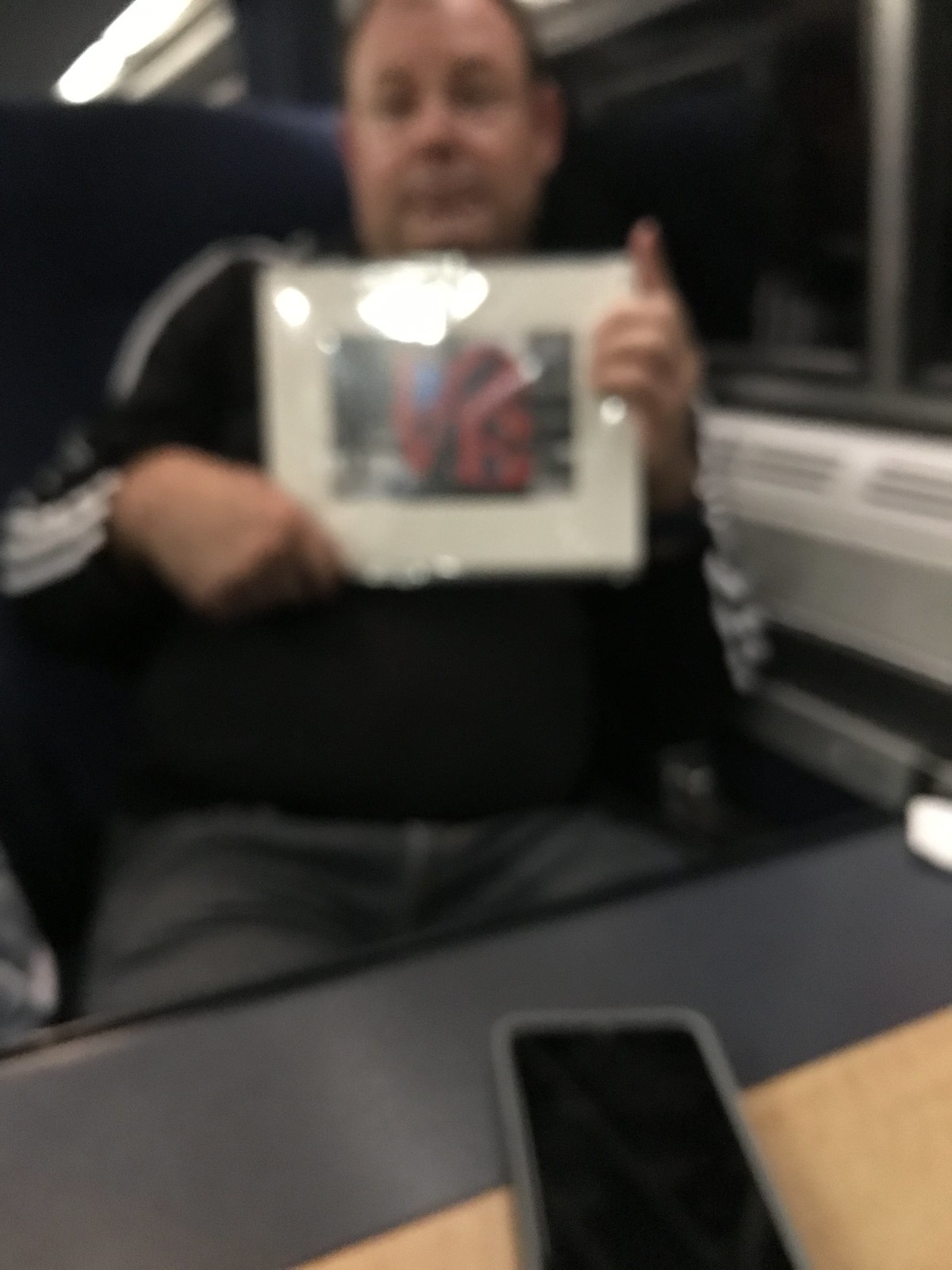In this blurry photograph, a portly, balding Caucasian man with dark hair is captured sitting on a train. He is wearing a distinctive black long-sleeve shirt with white stripes along the sleeves, resembling an Adidas tracksuit, paired with black denim pants and a black belt. The man holds an unidentified framed picture with a reflective, shiny white border, showing hints of red, green, and blue colors amidst the blur and plastic wrapping. He presents the picture with both hands, facing the camera, while maintaining a neutral expression. In front of him, on the tray table, lies a smartphone with a dark case and an inactive screen. The table itself transitions from a dark surface close to him to a light brown wood at the bottom right corner. Behind the man, additional lighting reflects off the window frame, which is silver, with venting alongside the white walls. The scene outside appears dark, indicating nighttime.